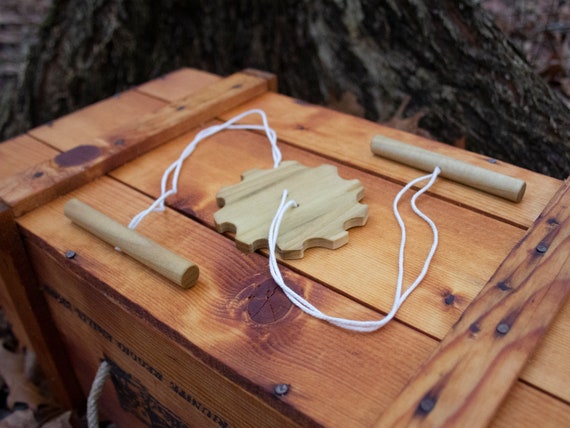This photograph features a natural, rough wooden box situated outdoors, as evidenced by the presence of a large tree trunk in the background. The box, appearing almost chest-like with visible wood knots and dark gray screws, has an unpolished, light-colored surface. A white rope-like handle extends from the front of the box, though the embossed words on it are illegible. On top of this box rests a handmade toy, comprising two light gray wooden cylinders connected by a white string. The string goes through both cylinders and features a circular, gear-like carving in the middle, giving the toy a rustic and playful appearance typical of a child's plaything.